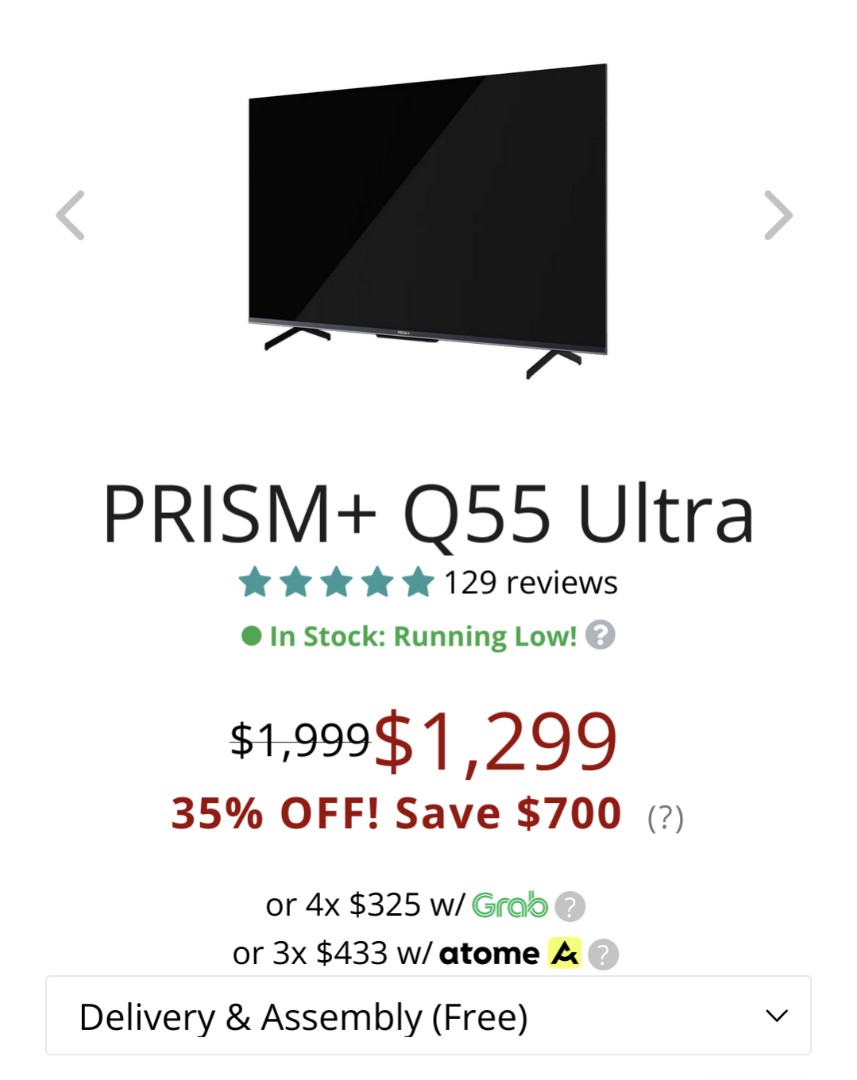**Caption:**

In the websites category, the webpage prominently features a flat-screen TV with a sleek, built-in stand. The TV screen is predominantly black, with a slight gradient suggesting light hitting it from an angle. Navigation arrows flanking the screen indicate the option to scroll through additional images. Beneath the TV is the model name, "Prism Plus Q55 Ultra," accompanied by a blue five-star rating based on 129 reviews. A green dot indicates that the item is in stock but running low. Further information can be accessed via a question mark icon. The original price of $1,999.00 is crossed out and replaced with a discounted price of $1,299.00, reflecting a 35% savings. Additionally, the product can be purchased through payment plans: four installments of $325.00 with Grab or three installments of $433.00 with Atomay. There's also an offer for free delivery and assembly.